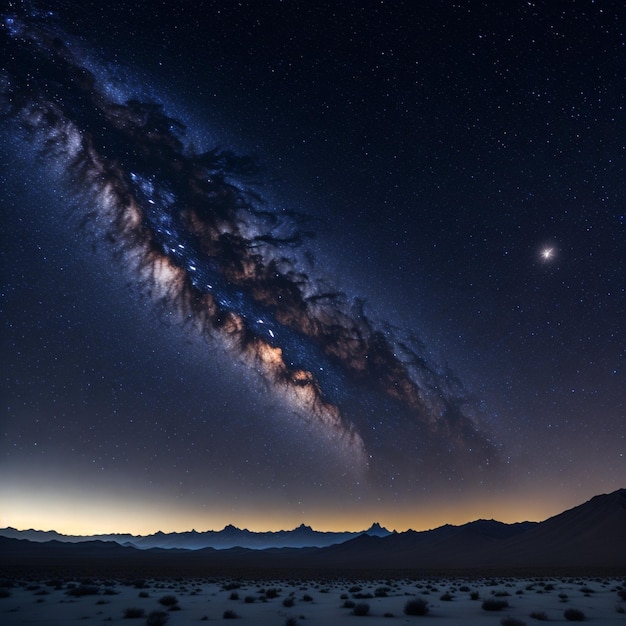The image showcases a mesmerizing night sky with an intricate play of colors and celestial objects. In the upper right-hand part of the image, a bright white light, likely the moon, illuminates the dark backdrop studded with countless tiny, white stars. Stretching diagonally from the upper left to the bottom right, a sprawling nebula or space cloud captivates with its glowing edges. The outer regions of this cloud shimmer in a bluish hue, transitioning to darker blue as you move inward, eventually blending into purples and oranges near the center. The core of this ethereal formation features specks of bright white light, resembling stars within a blue-tinged sky.

Below this cosmic display, the earthly terrain comes into view. The bottom of the image reveals undulating mountains, tinted with a soft, yellowish glow above them, hinting at twilight or moonlight. In the foreground, a desert-like expanse with sparse brush gives way to darker rock formations or dunes, creating a layered landscape. The overall scene exudes a sense of depth and surreal beauty, accentuated by the stark contrast between the celestial and terrestrial elements. The lower horizon is tinged with a lighter tan to brown shade, enhancing the whimsical yet dark ambiance of this stunning vista.